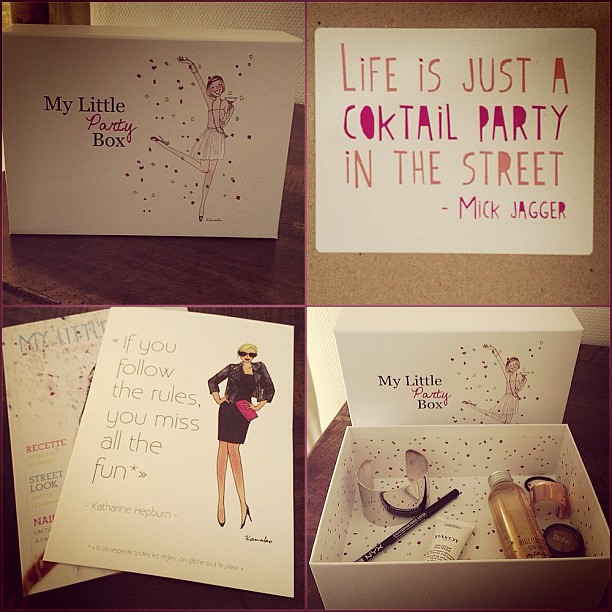This photograph features a product called "My Little Party Box," presented in a collage of four equally sized squares, two by two. Each square showcases different elements of the box and its contents. 

In the top left, a white box with "My Little Party Box" written on it is displayed, accompanied by a cartoon illustration of a woman throwing confetti while holding a martini glass. This scene rests on what appears to be a wooden table.

The top right square features a quote by Mick Jagger, "Life is just a cocktail party in the street," printed on white cardstock with pink lettering, seemingly mounted on a corkboard-like surface.

In the bottom left, another quote, "If you follow the rules you miss all the fun," by Catherine Hepburn, is depicted on a card. This card also includes a cartoon drawing of a woman in a black leather jacket over a black dress, high heels, sunglasses, and holding a pink clutch.

Finally, the bottom right square reveals the open "My Little Party Box," exposing its contents: a silver bracelet, black eyeliner, a tube of makeup, and several other small beauty products. The overall style of the image radiates a sense of fun and celebration, with varied colors including browns, blacks, pinks, whites, and golds.